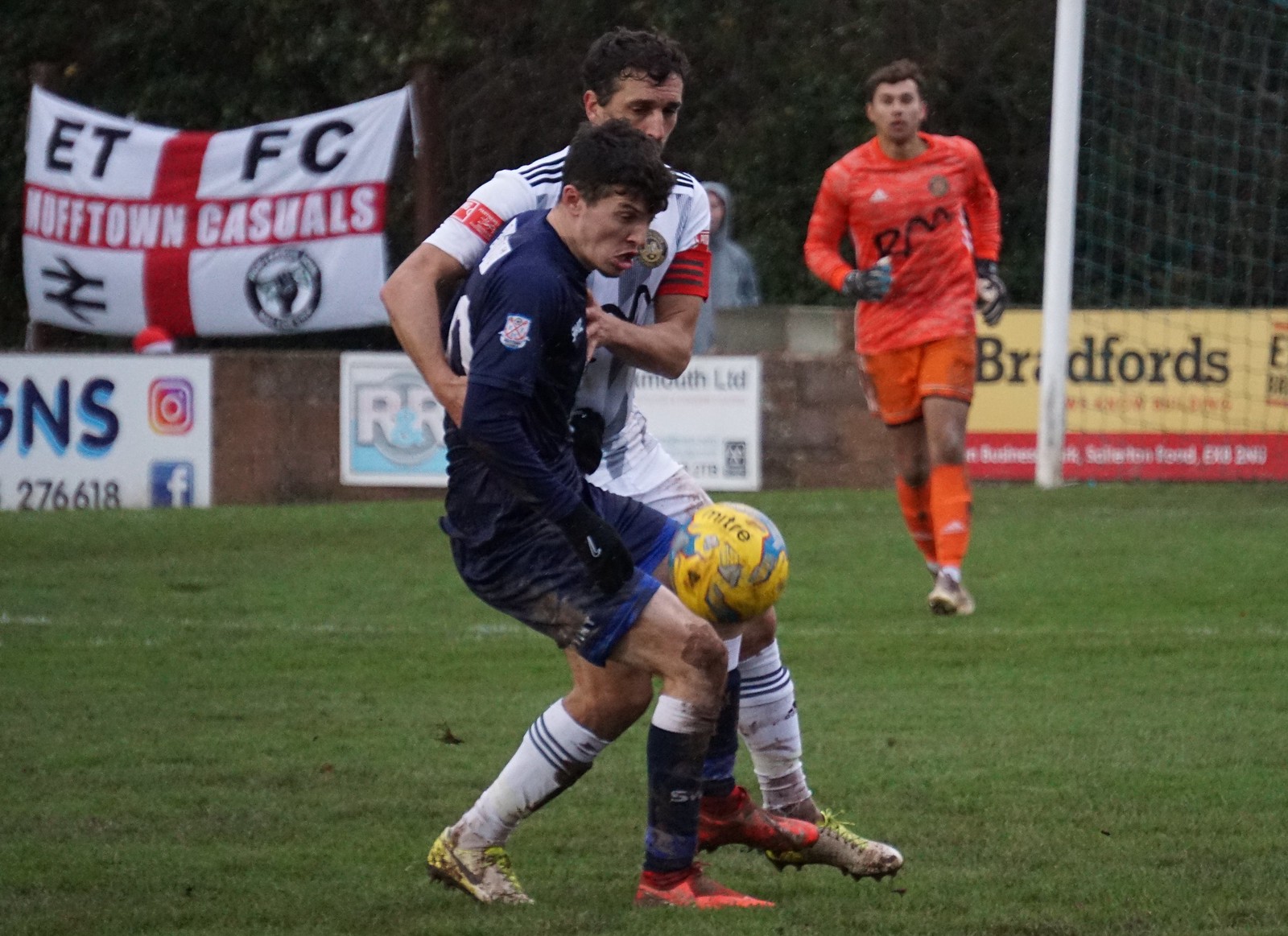The image captures a lively soccer match in mid-play, featuring three main players in dynamic action. Central to the scene, a player in a navy blue uniform, comprising a long-sleeved shirt, shorts, and black gloves, is intensely focused on a yellow ball positioned near his knee, his mouth open in concentration. Directly disputing the ball is another player dressed in a white uniform, accented with red and navy stripes. Both are on a lush, green grass field, their boots muddy from play. Slightly behind and running towards the action is a goalkeeper clad entirely in orange – jersey, shorts, and socks – suggesting a high level of engagement in the game. The background reveals a white goal net and boundary barricades adorned with sponsorship information, including one prominent banner reading "ETFC" and another stating "MDFF Town Casuals" along with logos and a phone number. A person in a gray hooded sweatshirt stands outside the barricade, observing the match. This daytime scene is rich in color and detail, encapsulating the vibrancy and intensity of a competitive soccer game.